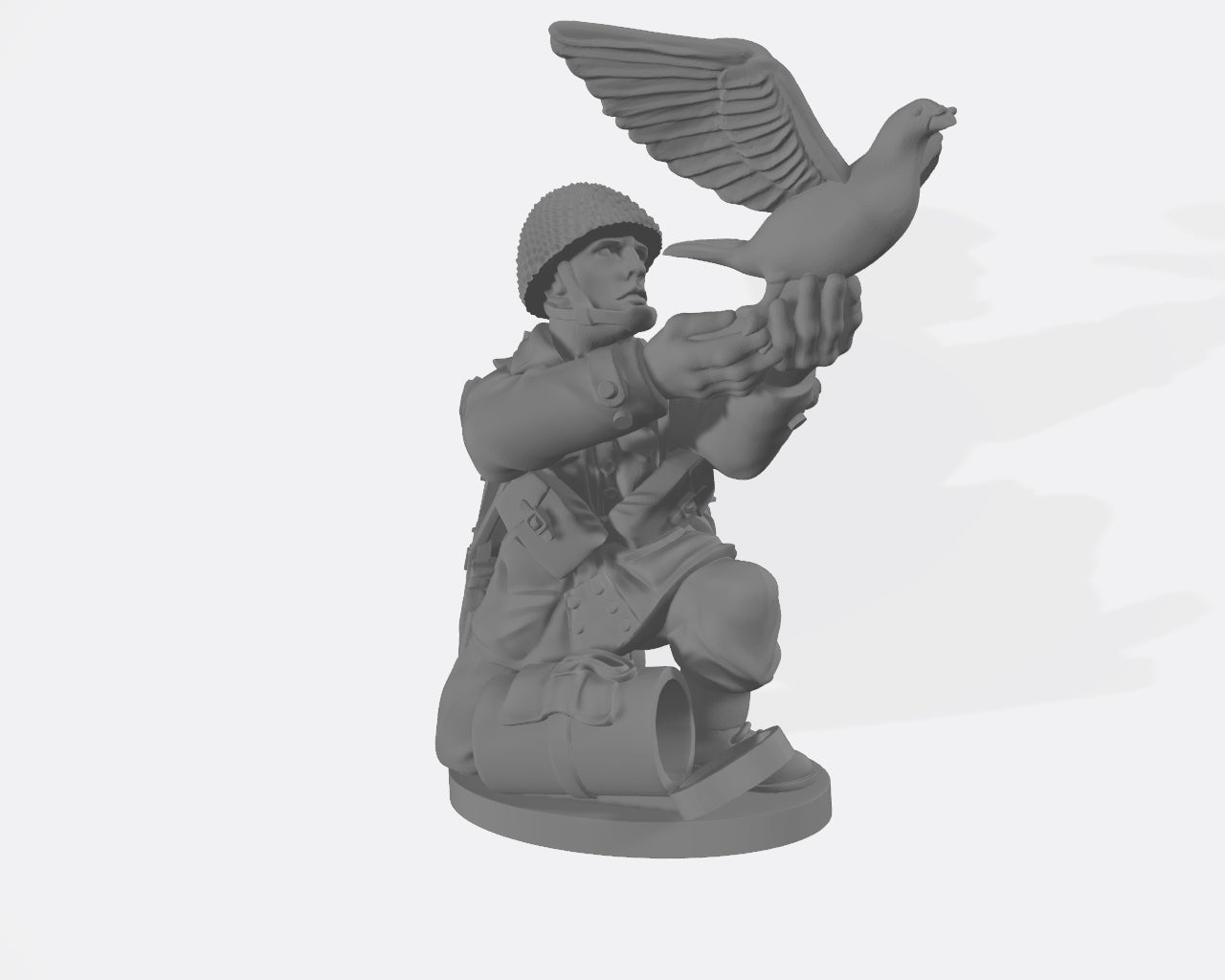This image features a detailed, antique gray clay sculpture of a kneeling soldier, central to the composition, depicted releasing a pigeon or dove into the air. The soldier, dressed in a uniform and helmet, sits on one leg with a cylindrical object, possibly a water bottle or bag, lying in front of him on the ground. The soldier's gaze is fixed upwards towards the bird, which is captured mid-flight with its wings fully extended. The entire scene, rendered meticulously in shades of gray, is set against a plain, light gray background that highlights the intricate craftsmanship of the sculpture. The image, devoid of any text, exudes a poignant sense of history and reverence.